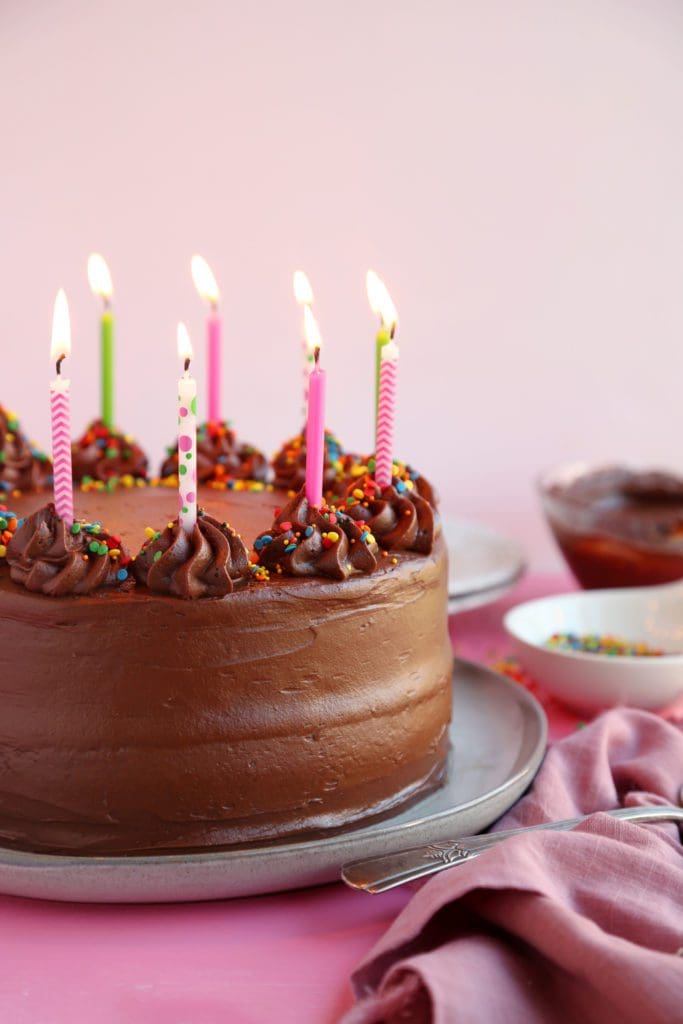This is a detailed close-up photo of a birthday cake set on a silver plate. The cake, positioned on a pink tablecloth, is delightfully covered in smooth chocolate frosting with intricate flower designs made from frosting, adorned with blue and green sprinkles. There are eight thin birthday candles visible, but the cake is partially cut off by the edge of the photograph, suggesting there may be more candles. The candles vary in color and pattern, including pink, white, green, and designs with red and white stripes or balloons.

In the background, there is a light gray wall and additional items on the table. On the bright pink tablecloth, a crumpled pink napkin in the lower right corner holds a piece of silverware, possibly a spoon or fork. Above this napkin, there is a white bowl filled with colorful sprinkles matching those on the cake, and further back, a clear bowl containing chocolate pudding. The entire scene is accentuated by the lively, lit candles casting a warm yellow glow, celebrating a festive occasion.